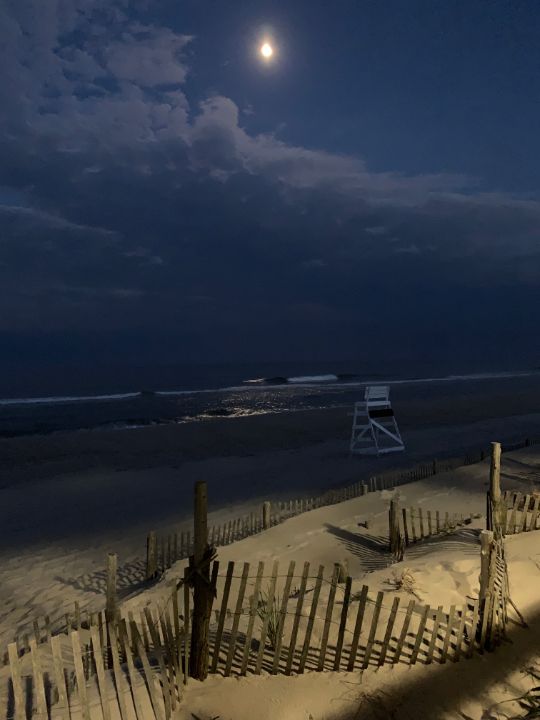A serene nighttime seashore scene is depicted with a luminous moon hanging in the sky, partially veiled by wispy clouds. The moonlight casts a silvery reflection on the gentle waves caressing the shore. Positioned slightly off-center to the right stands an elevated lifeguard station, crafted from white wood, its structure crisp against the night sky. Further back, a wooden fence likely marks an entrance to a walkway leading down to the deserted beach. There is a powerful light source emanating from the right side of the image, possibly from a nearby residence, illuminating the water with a brilliance that contrasts with the moon's softer glow. The beach lies tranquil and empty, inviting contemplation.